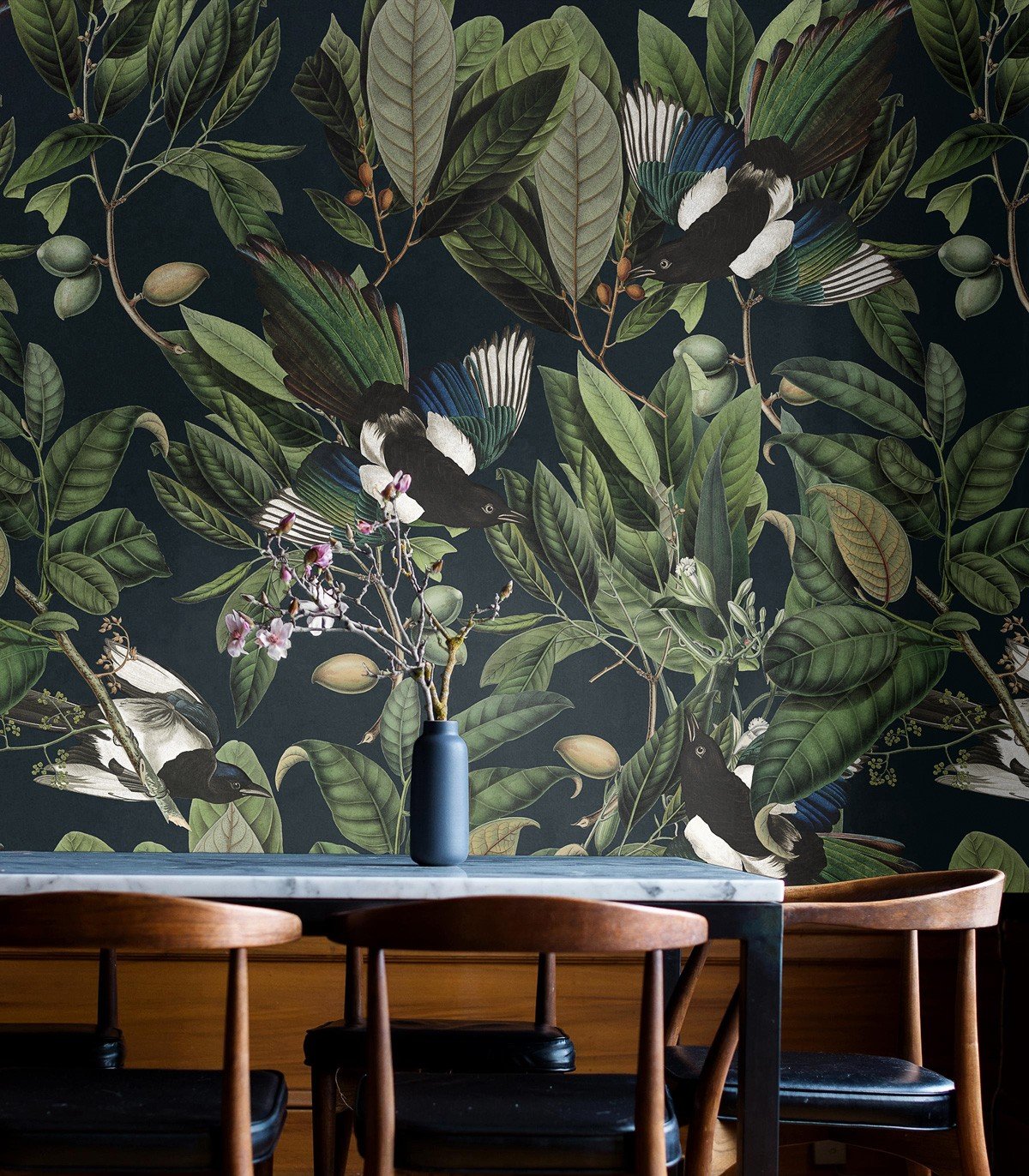This photograph showcases a stylish indoor space, possibly a coffee shop or a dining area, taken in portrait orientation. The main feature is an ornate wallpaper with a navy blue or black background adorned with intricate tree designs featuring large green leaves, which may resemble olive branches or mango trees, along with scattered seeds. Birds in flight, predominantly black with white, blue, and green wings and tails, are interspersed among the foliage. In front of this detailed wallpaper sits a long table with a white, marble-like tabletop and black metal legs. Surrounding the table are at least five wooden chairs with black leather seats. Atop the table is a black vase, tall and bottle-like, containing pink flowers and some sticks, adding a touch of organic elegance to the scene.